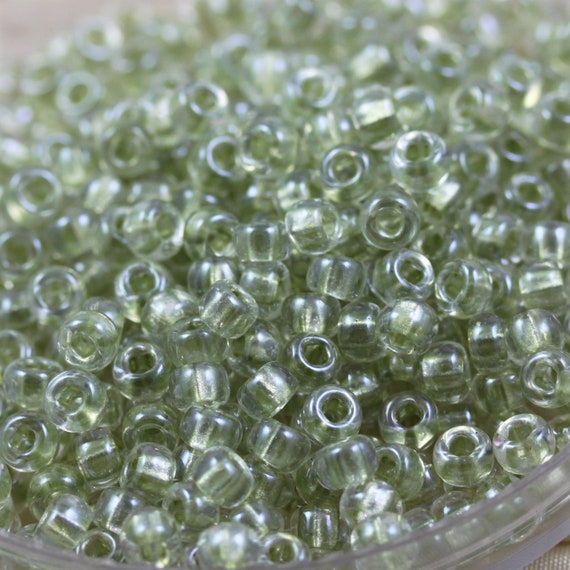This photograph captures a substantial collection of small, translucent, slightly greenish beads, densely piled within a large, clear plastic bowl. The beads, which are round with holes through the center for stringing, are numerous, numbering easily in the hundreds or perhaps thousands. The primary focus of the image is on the lower portion of the pile, with beads becoming blurrier towards the perimeter. The clear beads take on a slight green hue, giving an overall greenish tint to the collection. The bowl itself is see-through, revealing the texture of what appears to be a fabric surface or tablecloth beneath it. The rim of the bowl is visible at the bottom edges of the photo, showcasing the thickness and depth of the bead pile.